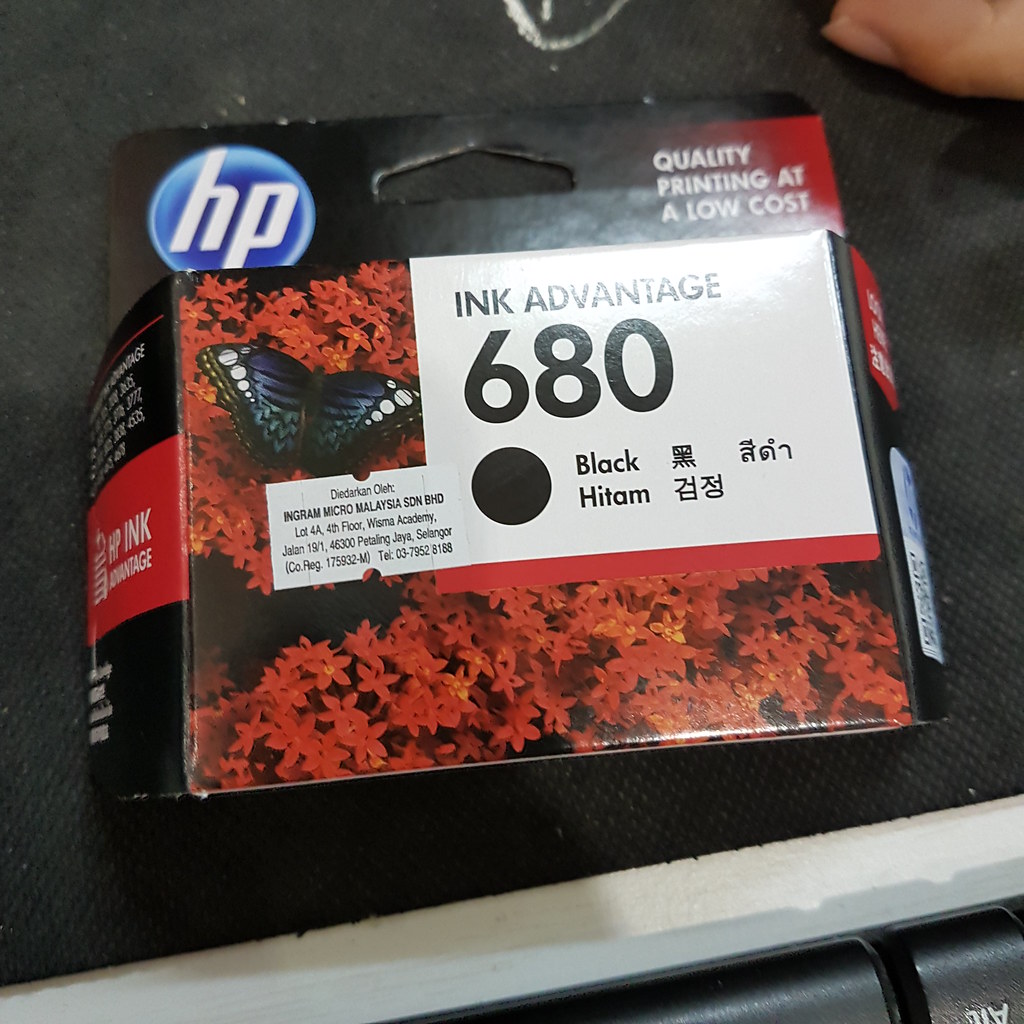This detailed color photograph captures a close-up of an HP ink cartridge box, resting on a black surface with white edges, possibly a mouse pad. Dominating the upper left corner of the box is the Hewlett-Packard logo, displayed as a blue circle with the white letters "HP" inside. In the upper right-hand corner, the phrase "QUALITY PRINTING AT A LOW COST" is prominently stated in white capital letters. The box itself, predominantly black, features a vibrant design of red flowers and a dark blue butterfly on the front, giving it a striking appearance. Central to the image, a white label reads "Ink Advantage 680" in bold black letters, with "BLACK" specified just below. Supplementary text, presumably in Malaysian, is visible but largely illegible due to size. Additionally, the photograph captures a small portion of a person's finger at the top right corner, adding a sense of scale and human presence to the image.